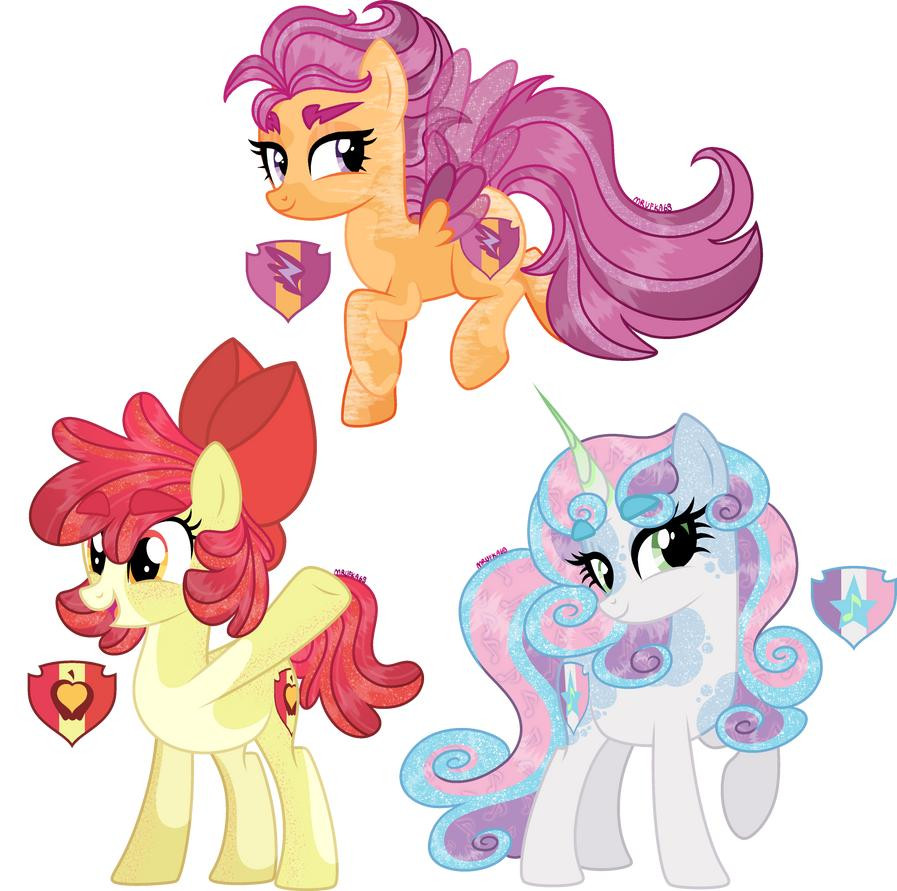This vibrant My Little Pony-style image features three distinct and colorful ponies arranged in a triangular formation on a white background. 

At the top of the triangle sits a tan pony with a flowing purple mane and tail. This pony sports little wings and has a distinct emblem on its hindquarter - a shield with light purple, yellow, and dark purple vertical stripes, adorned with a central lightning bolt. It also features purple eyebrows and light purple eyes accentuated with heavy eyeliner and long eyelashes.

The pony at the bottom left of the triangle is a pale, blonde-colored pony with a striking red mane, red tail, and a large red bow in its mane. This pony is depicted standing on three legs with its fourth leg raised, adding a dynamic element to its pose. Its eyes are orange and yellow, and it displays a similar shield on its flank with red, yellow, and red vertical stripes, but with a heart emblem in the center.

Finally, the bottom right corner of the triangle features a light purple pony with a mane and tail in shades of pink, sparkly blue, and purple. This pony is distinctive with a unicorn horn and light blue-purple splotches resembling clouds across its body. The mane's pink segments are further decorated with small musical notes, enhancing its whimsical appearance. Its shield has purple, gray, and pink vertical stripes, with a blue star and a green musical note in the center. 

Together, these three ponies create a lively and detailed composition, each bringing their unique features and emblems to the image.